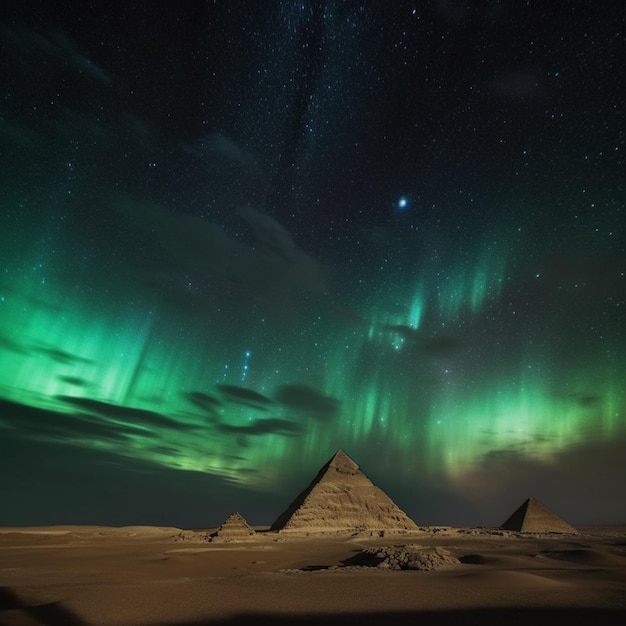This captivating photograph, which looks almost computer-generated, features a stark desert landscape in the foreground, characterized by flat sand and a small mound of rocks or ruins. Central to the image is a trio of the iconic Egyptian pyramids, with the tallest pyramid positioned in the exact center. To its immediate left is the smallest pyramid, both appearing relatively equidistant from the viewer, while the second tallest pyramid recedes into the distance on the far right. Above this timeless scene, the sky presents an awe-inspiring display: streaks of green aurora borealis light flow horizontally from the left to the right, creating a vibrant contrast against the night sky. A smattering of white stars punctuates the dark expanse above, including a particularly large, glowing blue star slightly right of center, approximately 75% up the photo. Illuminated blue lights also twinkle within the aurora itself, enhancing the surreal beauty of the night. Dark gray clouds add depth to the sky, anchoring the luminous spectacle above the ancient pyramids.